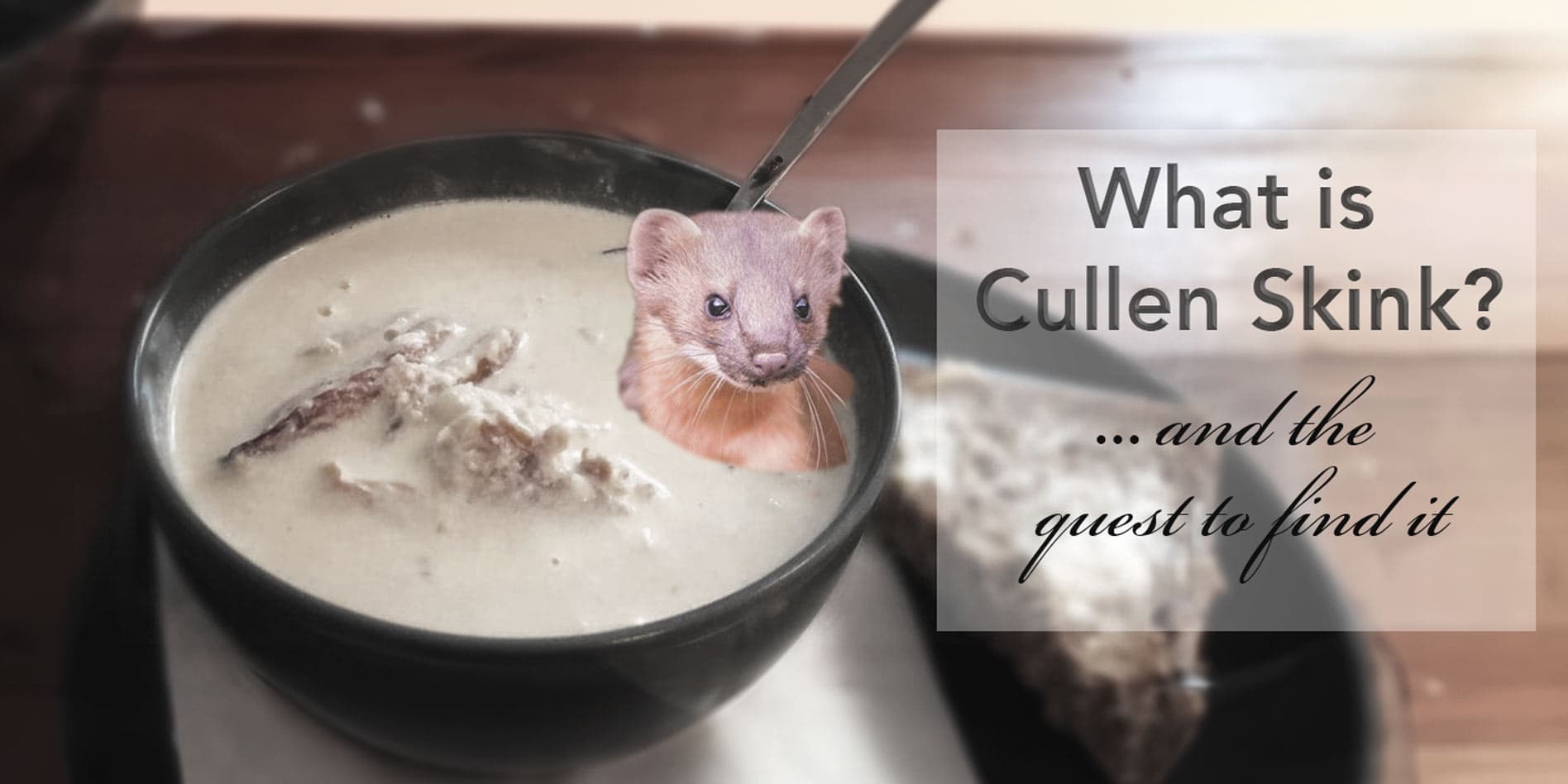The image features a whimsical food scene set against a brown table. At the center is a black circular plate holding a bowl filled with a white, soup-like substance, reminiscent of oatmeal or porridge. Emerging from the bowl is the head and neck of an ermine-like creature, brown in color, giving the impression it is dipped in the soup. A grey spoon is also inside the bowl. The bowl sits on a white tissue paper, and there's a triangular piece of toast placed next to it on the same plate. To the right side of the image, there is a text box with a translucent, whitish background formed into a square shape. The text intriguingly reads, "What is Cullen's skink and the quest to find it," inviting curiosity about the scene.